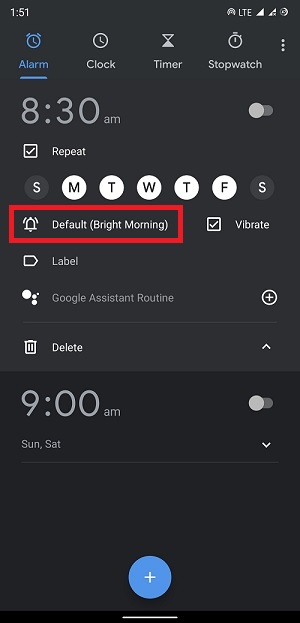The image depicts the settings screen of a smartphone alarm clock app, showcasing various alarm options and configurations. The screen is predominantly black with reverse print, enhancing readability. At the top left, the current time is displayed alongside hotspot and Wi-Fi icons. 

The app offers four distinct options displayed horizontally: Alarm, Clock, Timer, and Stopwatch. The "Alarm" tab, highlighted in blue, is currently active. Below this tab, an alarm is set for "8:30 AM" but is disabled, indicated by a slider button positioned to the left. 

Underneath the time, there's a checkmark next to "Repeat," and days of the week are shown with white circles for Monday to Friday and black circles for Saturday and Sunday, suggesting that the alarm is set for weekdays only. 

A red box surrounds the “Default: Bright Morning” sound option, indicating the tone the alarm will use. Adjacent to this, a checkmark beside "Vibrate" ensures the phone will vibrate when the alarm activates. 

Further down, there is an option to label the alarm and add a Google Assistant routine via a plus button on the right. A delete option for the alarm is represented by a trash can icon. 

Additionally, another alarm is set for "9:00 AM" for weekends (Saturday and Sunday), 30 minutes later than the weekday alarm. Users have the option to delete this alarm as well.

At the very bottom of the screen, there's a blue plus button for adding new alarms. To the right of the "Stopwatch" tab, three vertical dots indicate additional settings options.

Overall, the screen is efficiently organized, allowing users to manage alarms with ease.